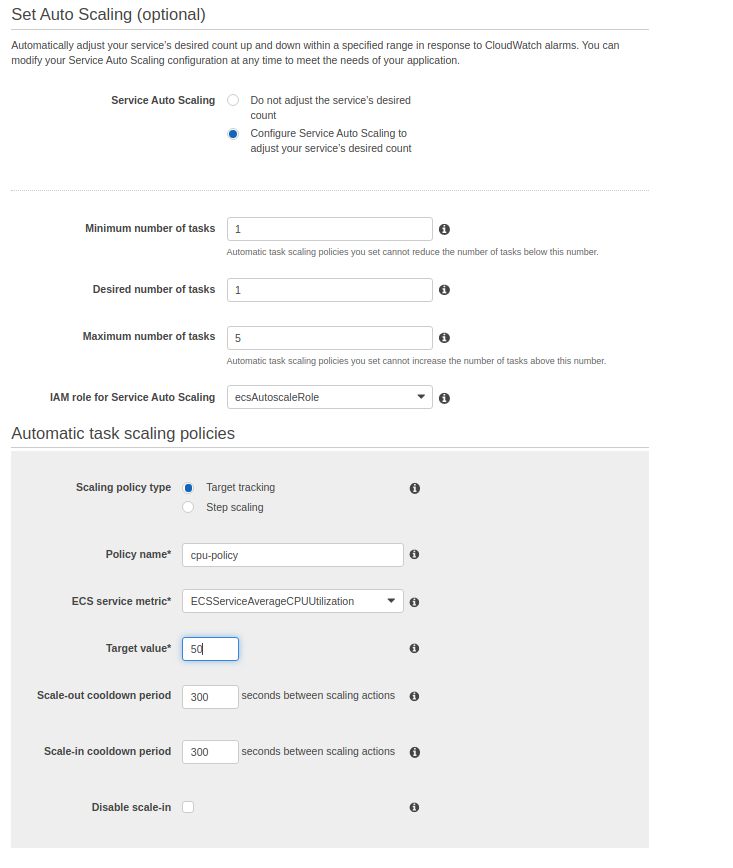The image depicts a webpage interface likely being viewed on a PC due to its sizeable layout, suggesting it isn't optimized for smaller devices like phones. The main heading reads "Set Auto-Scaling" with an indication that this feature is optional. Below this, there is an explanatory text stating: "Automatically adjust your service's desired count up and down within a specified range in response to CloudWatch alarms. You can modify your service auto-scaling configuration at any time to meet the needs of your application."

Indented underneath, there are two selectable options for service auto-scaling: 
1. "Do not adjust the service's desired count."
2. "Configure service auto-scaling to adjust your service's desired count." 

The latter option is highlighted in blue, indicating it has been selected.

Next, there are input fields specified for the following parameters:
- Minimum number of tasks: 1
- Desired number of tasks: 1
- Maximum number of tasks: 5 

Each parameter field features a black circle icon with an "i" symbol for additional information.

Further down, there's a section labeled "IAM Role for Service Auto-Scaling," which is set to "ECSAutoscaleRole."

Below this, the interface displays settings for "Automatic Task Scaling Policies," including:
- Scaling Policy Type
- Policy Name
- ECS Service Metric (with a drop-down box for selection)
- Target Value
- Scale Out Cool Down Period
- Scale In Cool Down Period

Each setting field has an accompanying information icon to provide more details. There is also an option to disable the scale-in feature, identified by a checkbox and an information icon beside it.